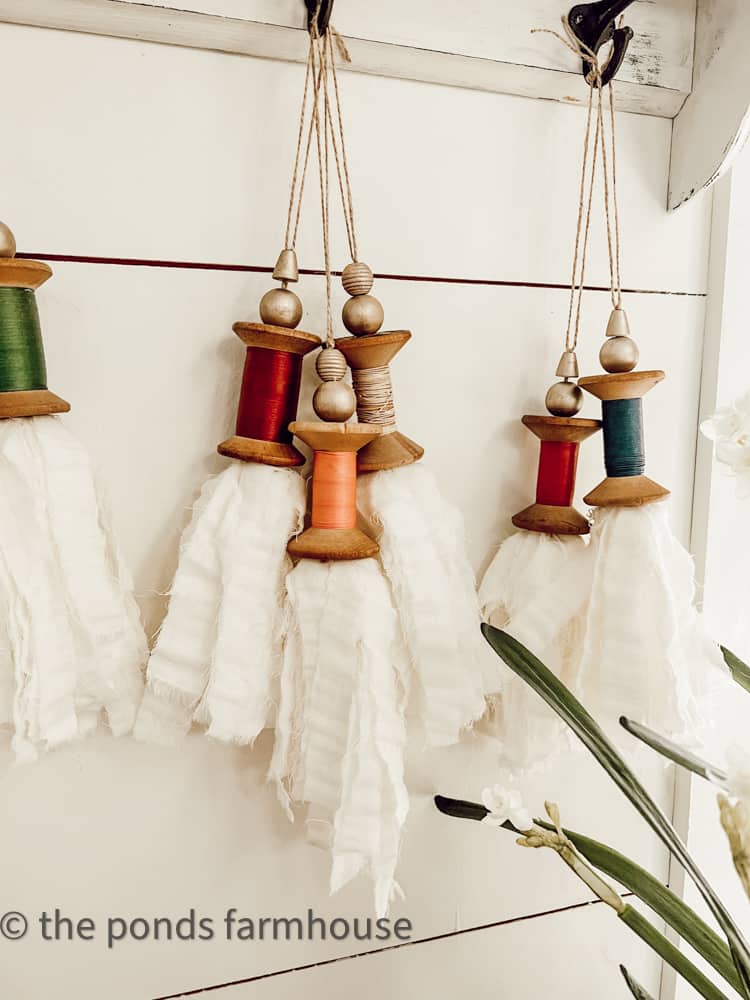The photograph captures a decorative arrangement inside a home, showcasing a white shiplap wall adorned with a mounted shelf featuring black metal hooks. From these hooks hang six wooden spools of thread, each detailed with delicate embellishments. The spools are connected by burlap strings to a sequence of beads - a triangular wooden bead followed by a round silver painted bead or a ridged bead variant. The color of the thread on each spool varies, including green, red, orange, peach, white, and blue, and from the bottom of each spool dangles crinkled white cotton fabric strips. The arrangement is both artistic and rustic, likely reflecting a farmhouse style. At the bottom left corner, a logo reads "copyright The Ponds Farmhouse," while the bottom right corner features a small plant with white flowers peeking into the frame.